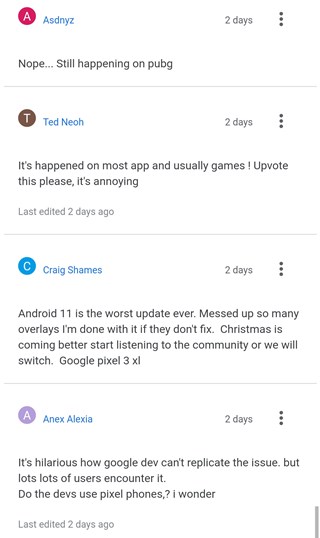Four users are engaged in a discussion on a Reddit thread about recent issues with Google devices, specifically Pixel phones. This conversation happened two days ago. The first user states, "Nope... still happening on PUBG," highlighting ongoing problems with the game. The second user responds, "It's happened on most apps and usually games! Upvote this please. It's annoying," indicating widespread issues and urging others to bring attention to the problem. The third user expresses frustration with Android 11, saying, "Android 11 is the worst update ever, messed up so many overlays. I'm done with it. If they don't fix it, Christmas is coming, better start listening to the community or we will switch," specifically mentioning the Google Pixel 3 XL. Finally, the fourth user adds, "It's hilarious how Google DEV Google maybe devices can't replicate the issue but lots and lots of users encounter it. Do the developers use Pixel phones, I wonder?" questioning the developers' understanding of the issue. The conversation underscores widespread dissatisfaction with a recent Android update affecting Google Pixel phones.